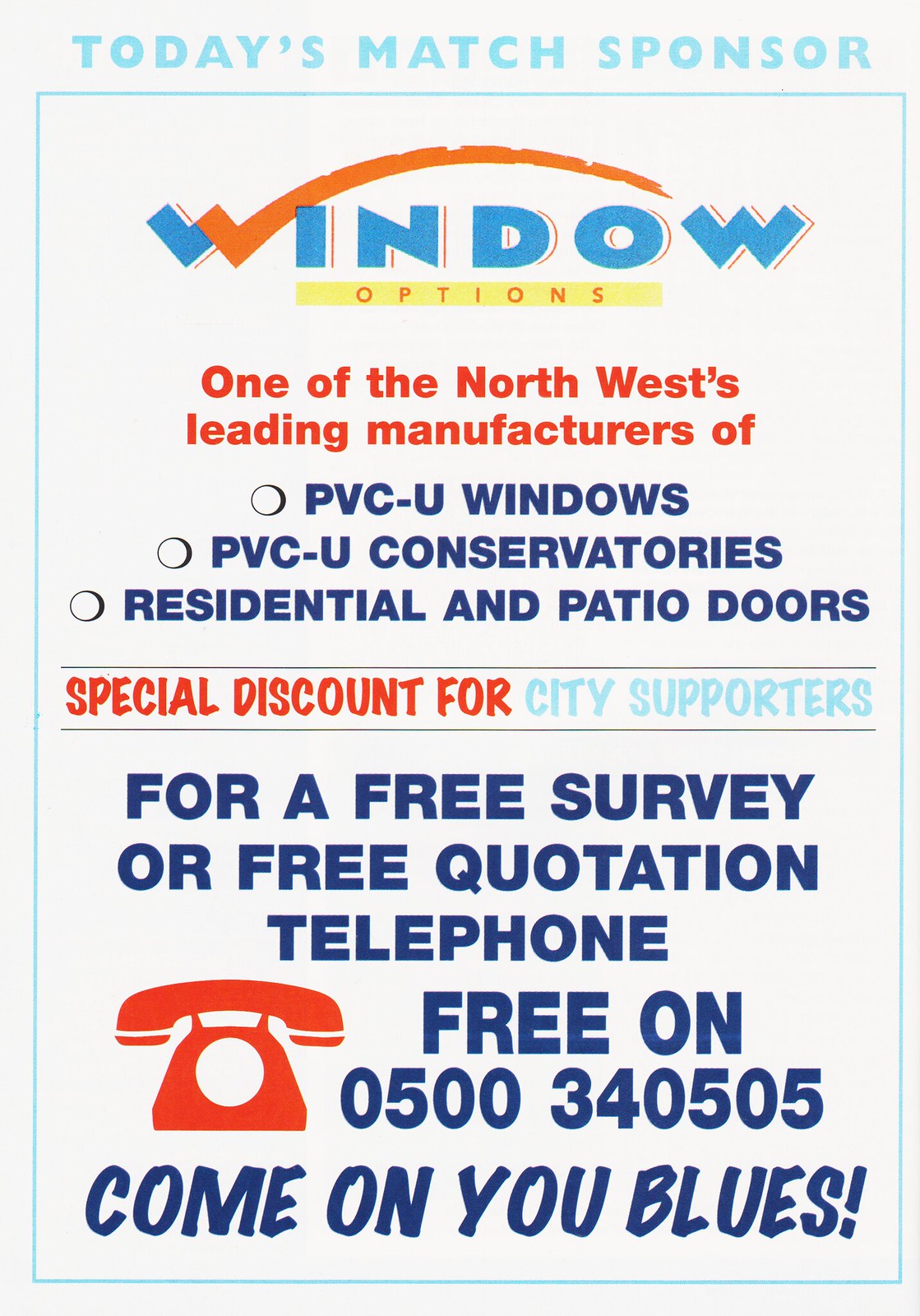The flyer prominently features the announcement "Today's Match Sponsor" at the top in light blue. Centered within a blue-bordered box, the primary text showcases the sponsor, "Window Options," a leading manufacturer in the Northwest known for PVCU windows, conservatories, residential, and patio doors. The brand's logo includes the word 'window' in white and blue capital letters, and 'options' in red, spaced-out lettering on a yellow rectangle. The flyer offers a special discount for city supporters and encourages contacting them for a free survey or quotation via a toll-free number, 0500 340 505. Additionally, the flyer features a small graphic of a retro corded phone, enhancing the invitation with "Come on, you blues!" at the bottom. The overall design is set against a gray-white background with a thin blue border framing the content.